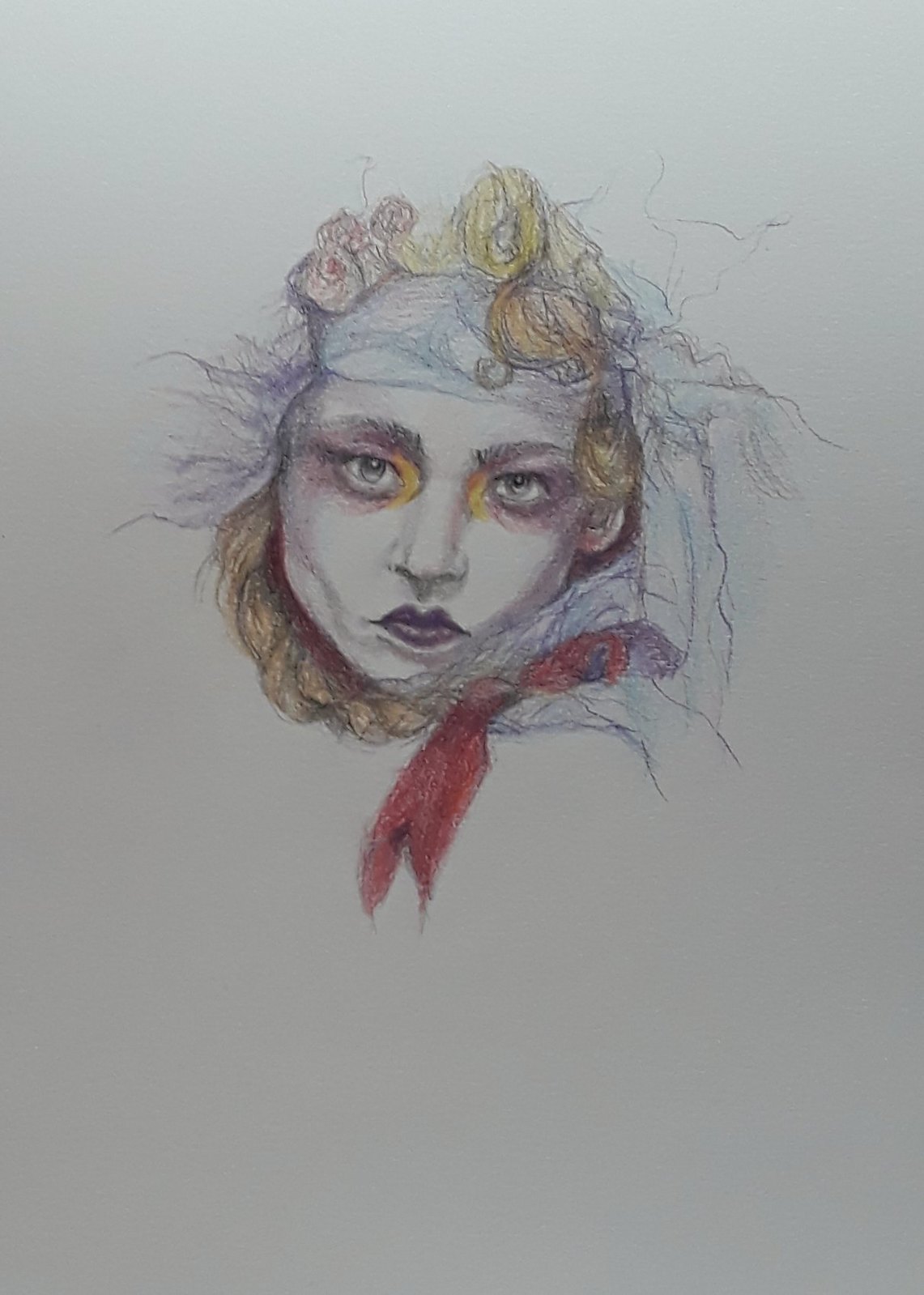This image captures an intricate and artistic drawing rendered with colored pencils. The subject of the drawing is a female face, expertly shaded with a striking emphasis around the eyes, where heavy makeup is depicted. The area beside the bridge of her nose features a soft application of yellow, adding depth and contrast to the complexion.

Her hair is long and styled with a feminine touch, partially braided beneath her ear on the left side, and draped elegantly below her chin. She adorns a vibrant headdress embellished with delicate flowers, adding an element of nature to her appearance. Strands of her hair are visible, extending around the top and back of her head, creating a soft, flowing effect.

Around her neck, she wears a scarf, gracefully wrapping around and appearing next to her chin on the right side of the image. The drawing exists on a plain white sheet of paper, with no other objects or details in the background, thus highlighting the intricate artistry and vivid colors of the portrait.